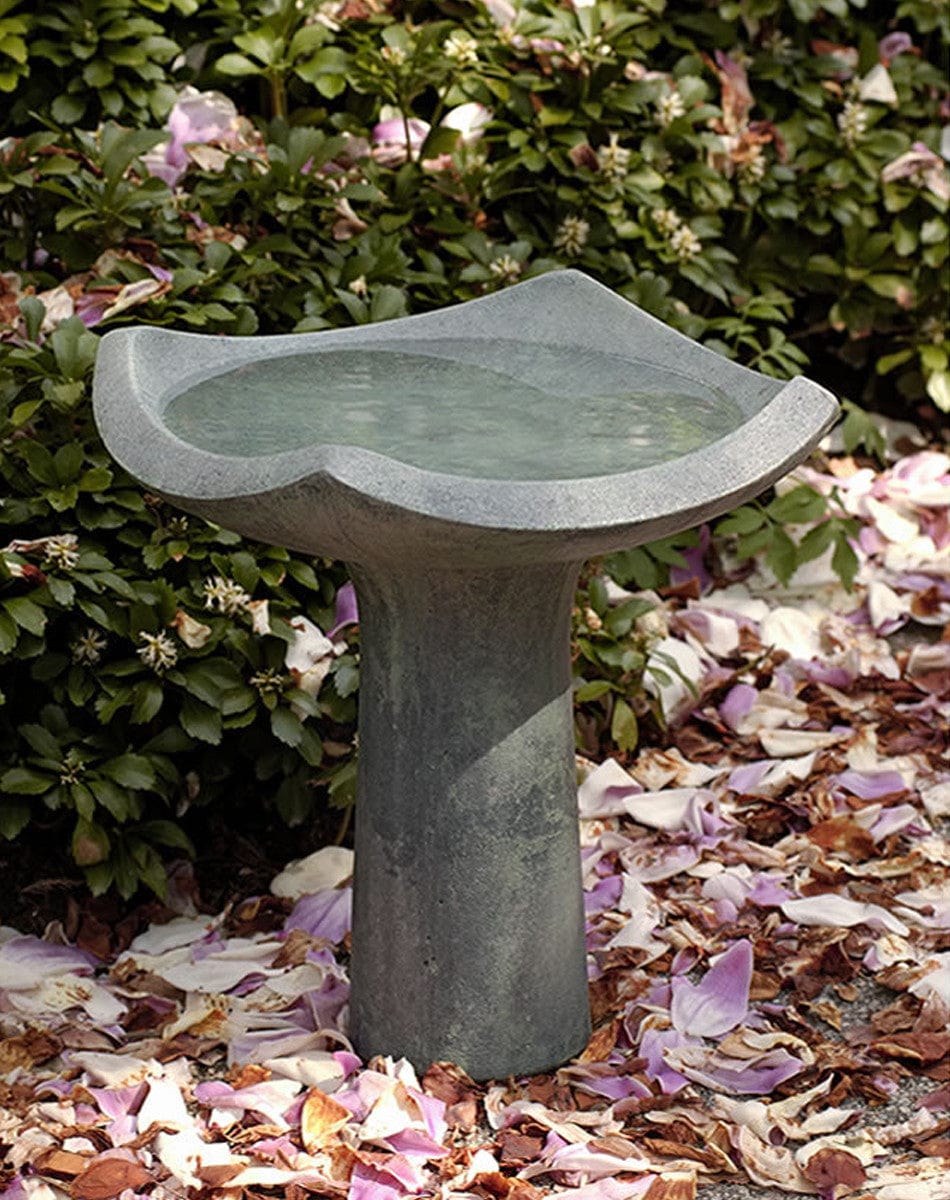The photograph depicts a serene, zen garden scene centered around a unique stone birdbath. The birdbath, crafted from concrete, features a wavy, four-sided design, resembling a flat square with its corners artfully curved upward to form a bowl. Seated atop a sturdy stone pillar, this birdbath is filled to the brim with water, ready for any bird to come and bathe. Surrounding the birdbath, the ground is scattered with fallen pink flower petals and brown, dead leaves, with the petals in various stages of decay. A large green shrub with a few remaining pink and purple flowers can be seen in the background, where most of its blossoms have already fallen. The entire scene is bathed in sunlight, casting a peaceful, warm glow over the setting, highlighting both the simplicity and tranquility of the birdbath and its natural surroundings.